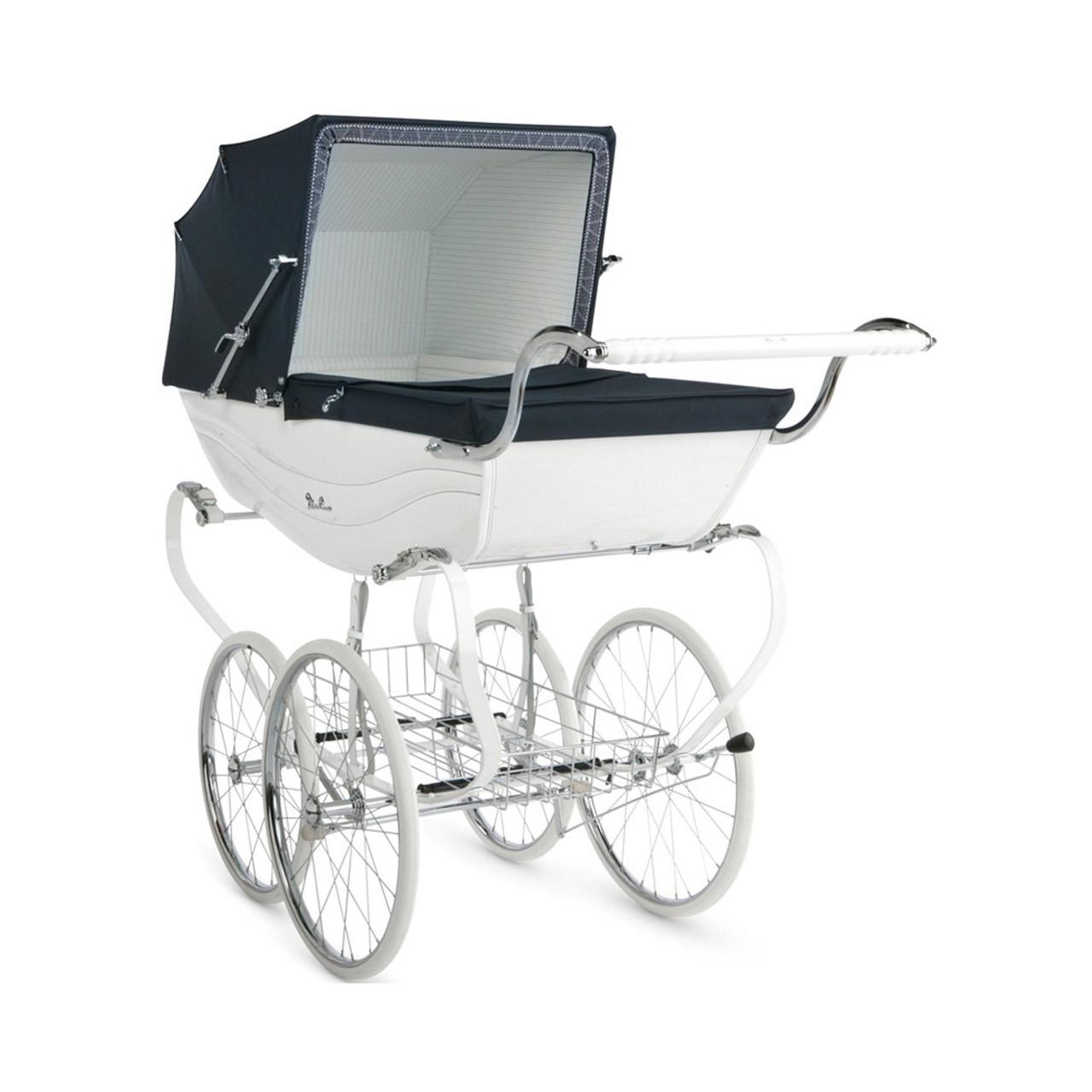The image depicts a high-end, ornate baby carriage with a vintage, retro design. The carriage features a luxuriously detailed chrome frame with elements painted in white, and it is supported by four large, white bicycle-like wheels with metal spokes. The frame’s design includes elegant curves that connect to a front handlebar. The carriage is topped with a black folding canopy that can be opened or closed, revealing a white cloth interior with a striped texture. The side of the buggy bears a silver logo, although it is too small to read. The photograph is taken from an angle facing the bottom right-hand corner, and it is set against a plain, white, transparent background, allowing the elaborate details and craftsmanship of the carriage to stand out prominently.